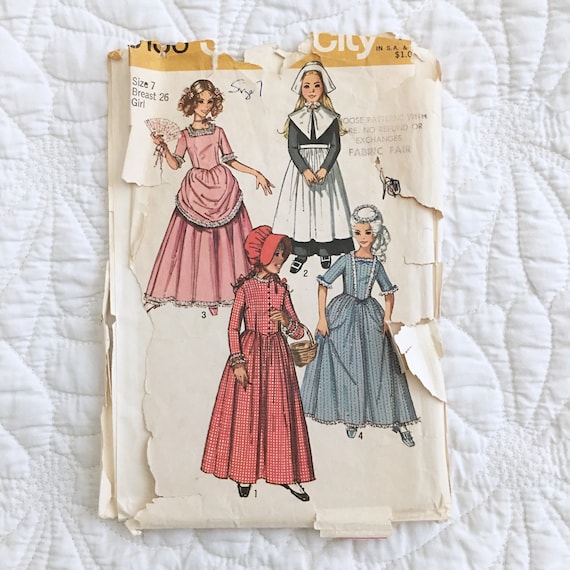The image depicts a vintage, heavily worn dressmaking pattern set atop a white quilted cloth background. The pattern, severely tattered at the edges with parts missing from the top and left sides, once bore a name now obscured by the damage. However, visible text indicates: "size 7, breast 26, girl." The pattern features illustrations of four young girls in distinct, historical-style dresses. One girl is depicted in a formal pink gown, holding a fan. Another wears an Amish or pilgrim-like outfit, characterized by dark fabric, a white cap, capelet, apron, and a sizable collar. A third girl is dressed in a red outfit reminiscent of Little Red Riding Hood, complete with a hood and a basket. The fourth girl resembles Marie Antoinette with her elaborate white hairstyle and blue-and-white striped formal gown. Each dress evokes a different era, encapsulating a diverse array of historical fashion styles.